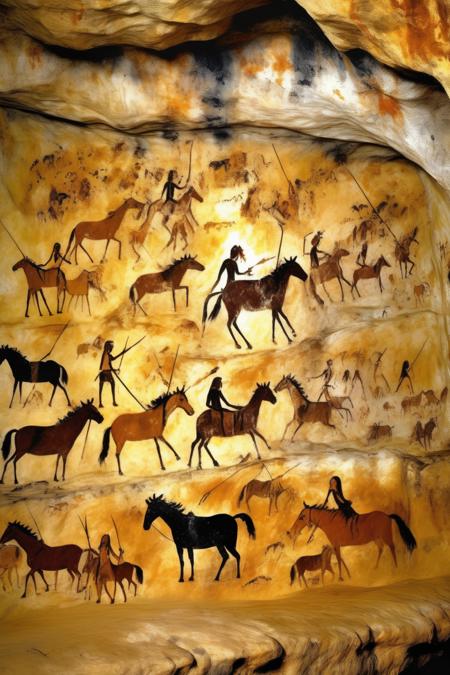In this detailed photograph or illustration of cave paintings, the scene is illuminated by artificial light, showcasing a vivid depiction of a hunting or domestication expedition. The cave wall and ceiling display a palette of earthy tones, including brown, gray, black, white, yellow, and tan. The artwork is arranged in three to four distinct rows or levels. The paintings primarily feature horses, some with riders holding spears and others without, alongside figures on foot who are similarly equipped with spears. These figures appear to be engaging in activities that reflect either hunting or the domestication and trading of horses, as suggested by their organized efforts to keep the animals in line. The imagery offers a rich narrative without any accompanying text, capturing the essence of the artist’s portrayal of tribal life.